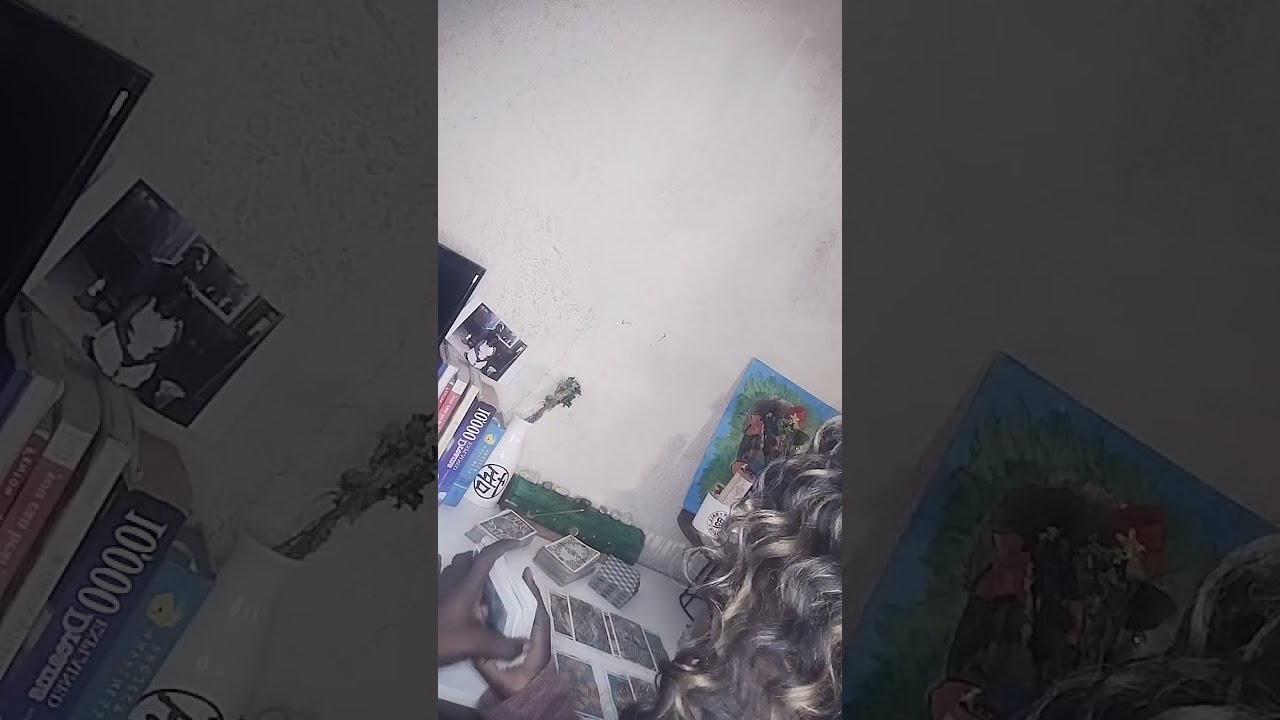The image is divided into three sections, with the central section being the brightest and serving as the focal point. In the center, we see the back of a person's head, characterized by curly brown hair with light streaks. This individual is seated at a white table, and their hands are visible above it. A pair of Black hands, belonging to the person, is holding a deck of cards. On the table to the right of their hands, multiple cards are spread out, accompanied by three additional decks of cards in front of the spread. Behind these cards, several books lean against a white, slightly dirty wall, one of which bears the title "10,000."

The left section of the image is a magnified view focusing on the books and the corner of a computer monitor. Above these books is a picture featuring a person's face. The right section, also magnified, shows the area just above the person's head, revealing a painting with blue, green, and brown hues. This section is dimmed, along with the left, to emphasize the detailed activity in the center.

In summary, the image captures an over-the-shoulder view of a person with curly brown hair engaged in card-related activity at a white table, surrounded by decks of cards and a stack of books, set against a slightly dirty white wall adorned with pictures and a piece of art.